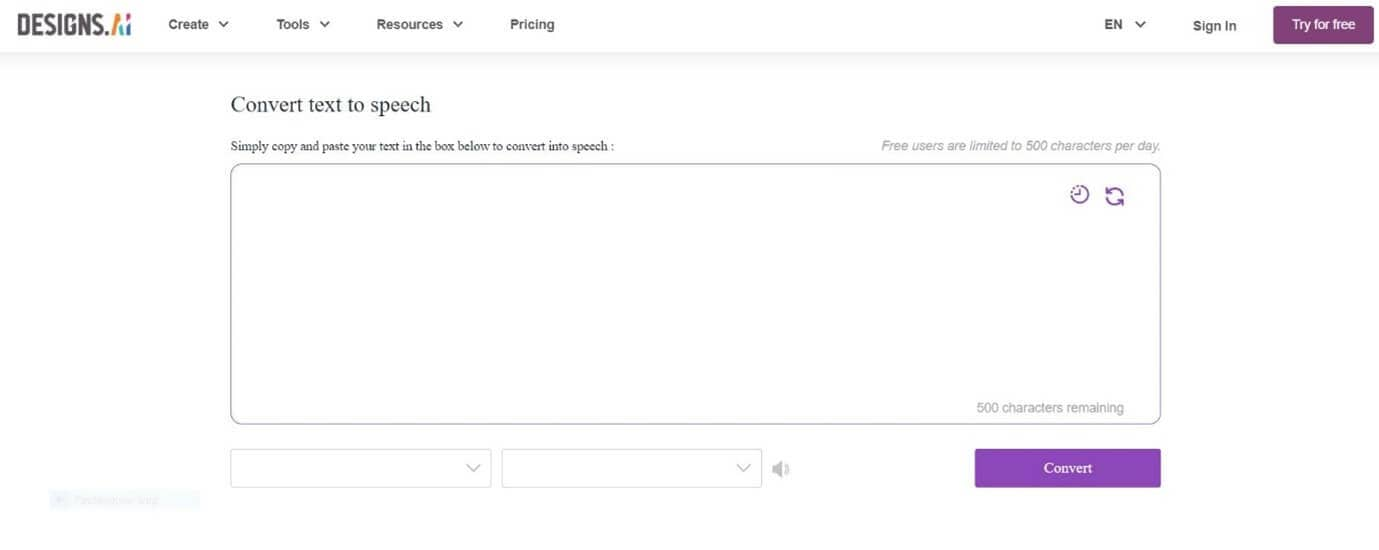The image features a user interface for a text-to-speech conversion tool. At the top, there are navigational options for "Designs," "Create," "Tools," "Resources," and "Pricing," alongside language selection "EN" and buttons to "Sign In" or "Try for Free." Below, a text box is designated for users to copy and paste their text, limited to 500 characters daily for free users. Adjacent to the text box is an icon of a clock and two arrows forming a circle, symbolizing the character limit. There are also two drop-down menus for additional settings, a speaker icon, and a prominent purple button labeled "Convert."